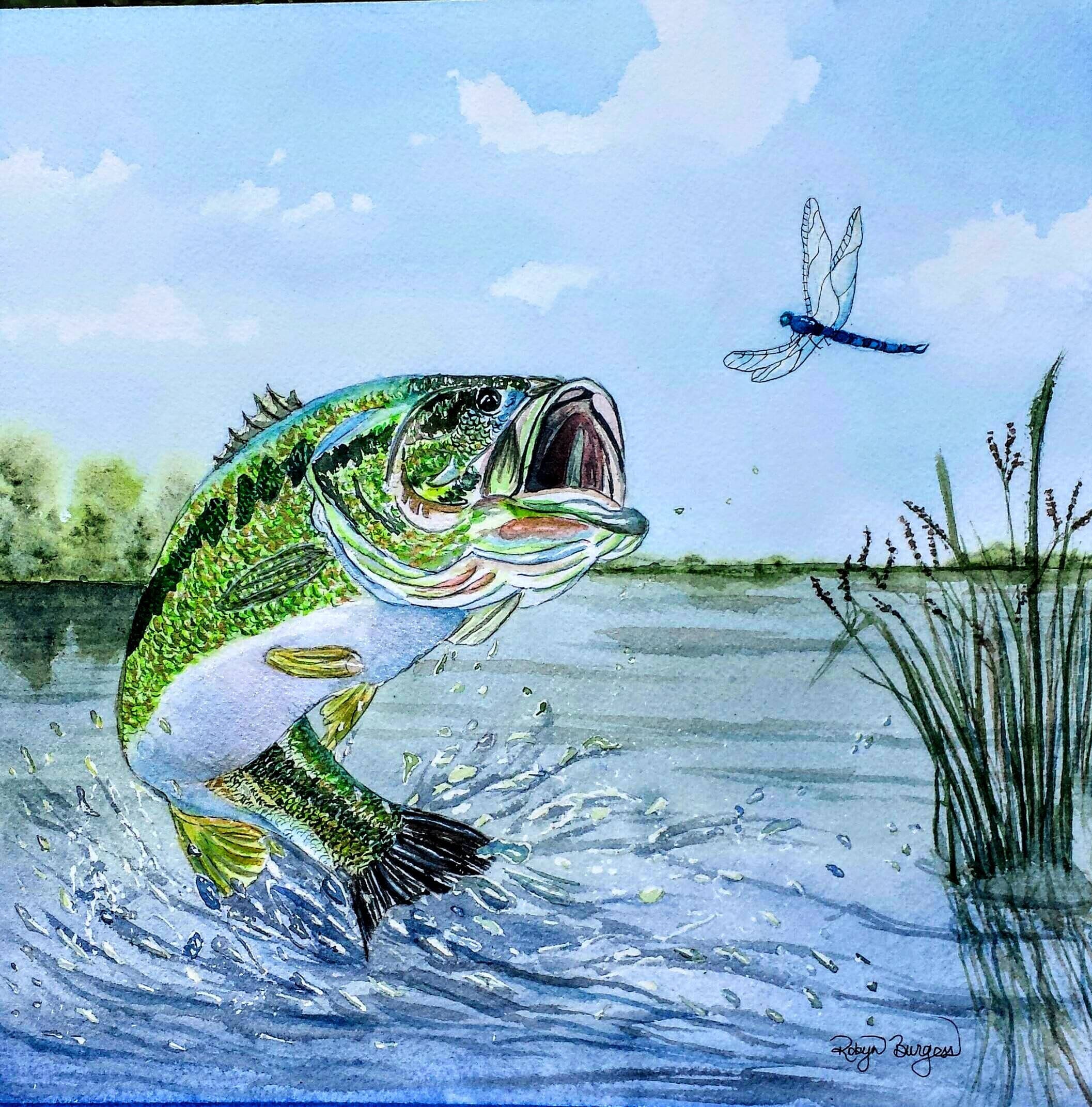This is a detailed watercolor painting depicting a lively scene of a fish leaping out of the water to catch a blue dragonfly. The fish, resembling a green trout or possibly a bass, has its mouth open and body curved with its tail still in the water, creating a dramatic splash. To the right, there are water reeds and tall grass with flowers, adding texture to the scene. The background features a forest of trees on the left and a flat plain on the right, with the reflections subtly casting shadows on the water. The sky is a vibrant blue with scattered clouds. The artist, Robin Burgess, has signed the piece in the bottom right corner. The painting's dominant hues are blues and greens, creating a harmonious and serene atmosphere.